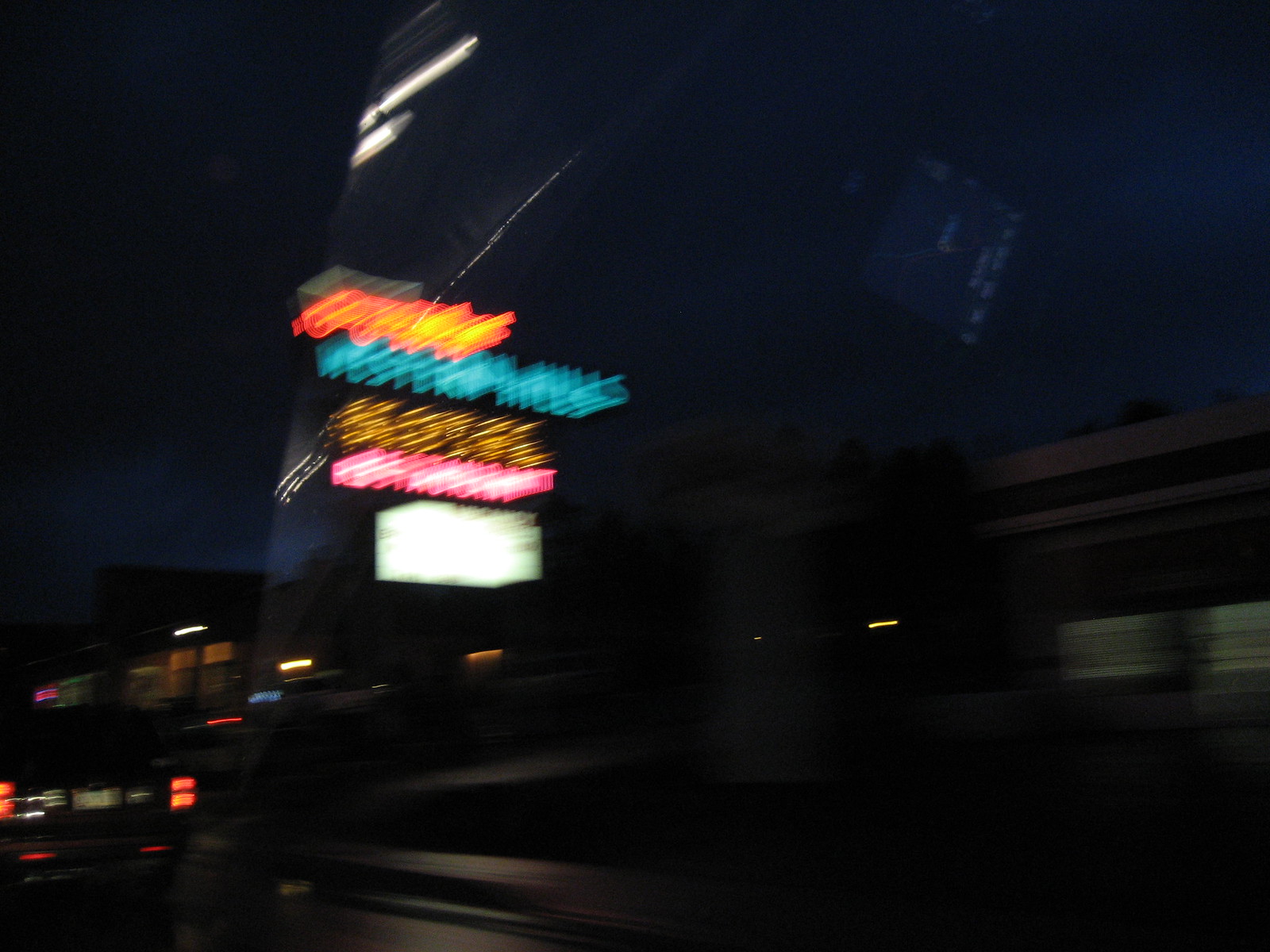This photograph captures a nighttime scene taken from a moving vehicle, resulting in significant blurriness due to the darkness and motion. The image reveals faint reflections from the vehicle window and some visible molding. In the adjacent lane, the red taillights of a car are discernible, indicating traffic beside you. The background features an establishment with a striking neon sign, displaying four words in distinct, vibrant colors: the top word is illuminated in orange, the second in aqua, the third in yellow, and the bottom word in pink.